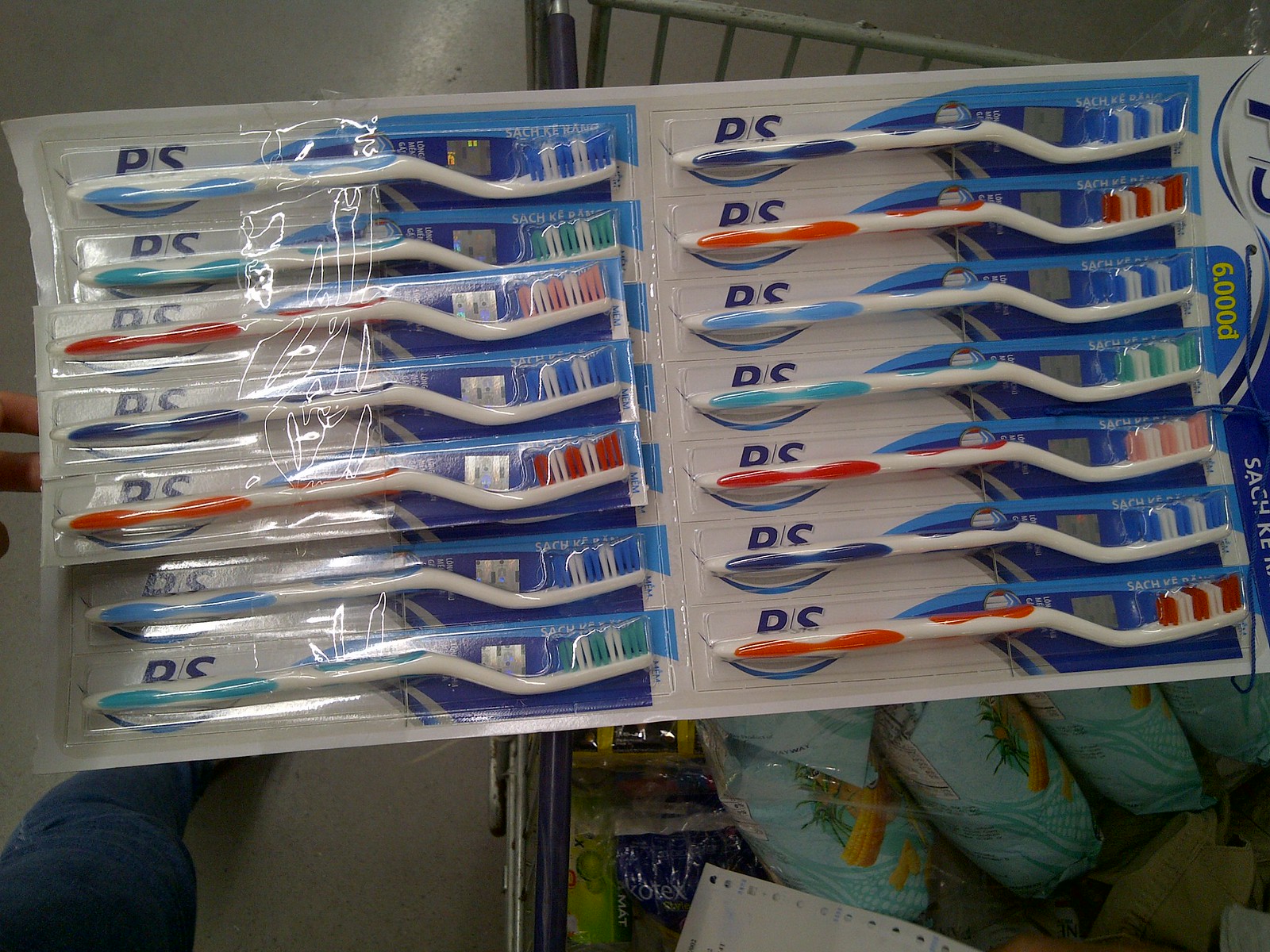In this indoor close-up color photograph, we see an economy pack of 14 individually plastic-wrapped toothbrushes arranged in two columns of seven on a white background with some blue striping. The toothbrushes are positioned with their heads pointing to the right and handles to the left. The colors of the toothbrushes include various combinations of blue, green, pink, red, and light green. The base of each toothbrush is marked with "PS," though this is partially obscured by the handles. At the top right corner of the package, we see the notation "6000 D PS," also slightly obscured. The lower part of the image hints at a shopping cart set against a background that includes what appears to be a rack, some pillows, and a piece of paper. There is also a blue light towel visible toward the bottom left corner, and part of a person's leg can be seen on the left side of the frame. The image is somewhat dark and slightly out of focus.